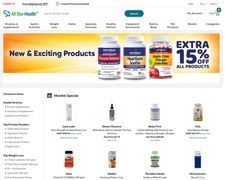A screen capture of a website dedicated to selling vitamins is depicted. The interface appears compact, making specific details challenging to discern. In the center, a prominent banner heralds "New and Exciting Products," accompanied by an image of three indistinct vitamin bottles. An enticing offer of "Extra 15% Off All Products" is also prominently displayed. The top portion of the site features a series of tabs likely designed to navigate to various categories of nutritional products. Below the main advertisement, the page showcases eight small vials, drops, and pill containers, though their exact contents remain indeterminable due to the image’s diminutive size.